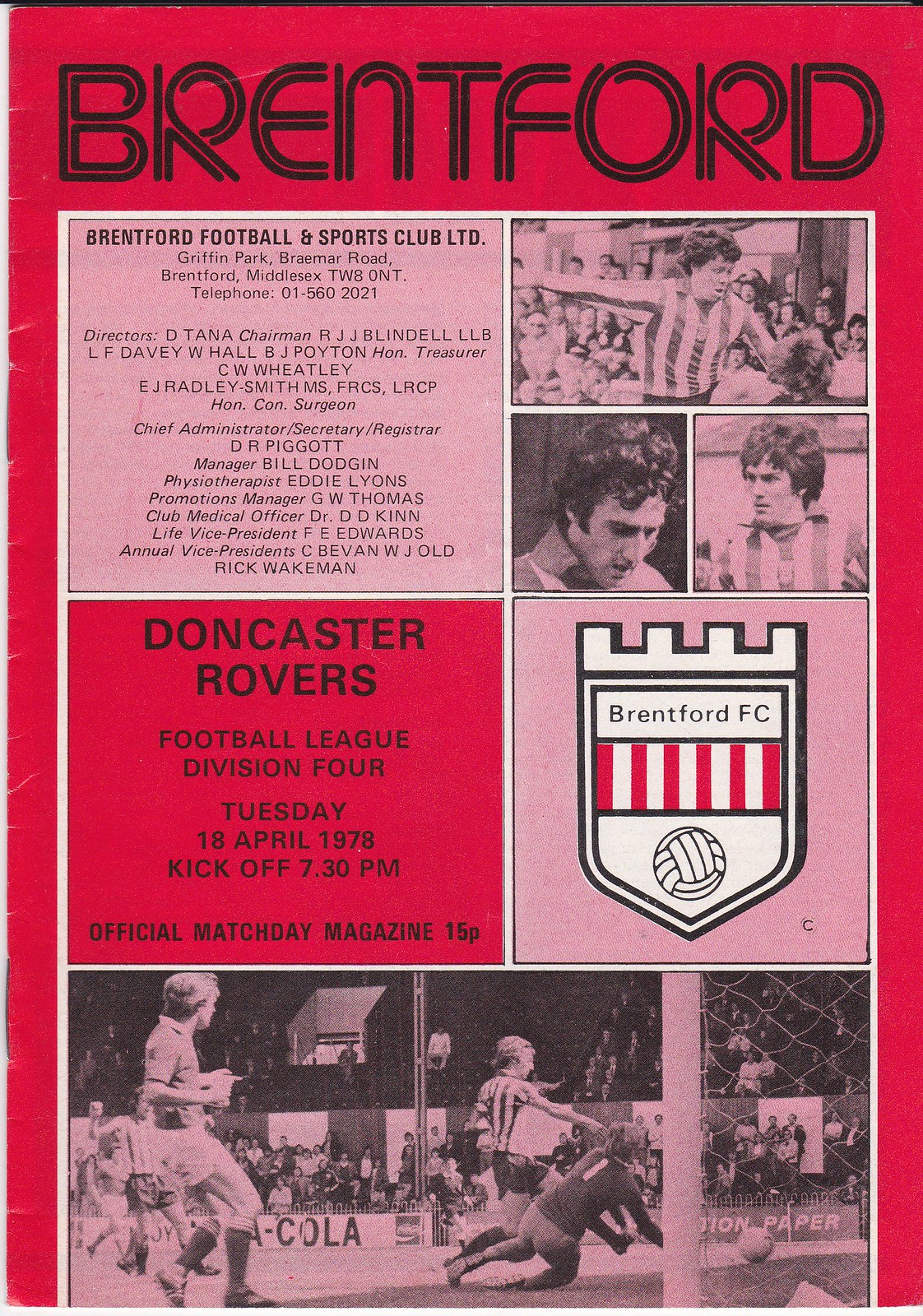The image is the front cover of an old-fashioned sports program, primarily featuring the Brentford Football Club. Dominated by bright red and light pink colors, the cover headline reads "Brentford" in black font on a red background. Below the title, a grid of light pink squares outlined in white includes detailed club information such as "Brentford Football and Sports Club, LTD," contact details, and the names of directors, promotions managers, and other officials. Prominently displayed is the Brentford FC crest, with red-and-white lines and a football symbol. Adjacent to the crest, a notable dark red box in black font announces the match: "Doncaster Rovers, Football League, Division 4, Tuesday, 18 April 1978, Kickoff 7.30 PM, Official Match Day Magazine, 15p." At the bottom, a pink box showcases an action shot of a soccer match in progress, with players moving towards the goalpost on the right.